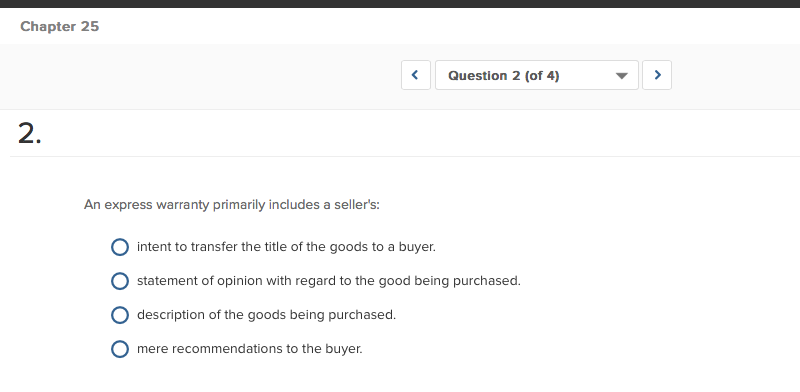**Detailed Caption:**

The top of the image features a medium black line serving as a border. Directly beneath this border, positioned towards the left, the bold gray text "Chapter 25" is clearly visible. Below this, a rectangular section with a light gray background extends across the frame. Towards the middle-right area of this section, there are two blue arrows—one pointing left and the other pointing right—each enclosed in square icons with light gray borders.

Centrally aligned within the rectangular section, a drop-down menu displays the bold gray text "Question 2 (of 4)." Transitioning from this area, the background shifts to white. In the upper-left corner of this white section, a dark gray number "2" followed by a period is visible. A faint gray thin line acts as a divider below this number.

The main content is a multiple-choice question, each possible answer preceded by a small circular radio button outlined in dark blue. The question posed is in black, small, basic sans-serif font, asking: "An express warranty primarily includes a seller's:" followed by a colon. The multiple-choice answers are listed as follows:
 
1. Intent to transfer the title of the goods to a buyer.
2. Statement of opinion with regard to the goods being purchased.
3. Description of the goods being purchased.
4. Mere recommendations to the buyer.

None of the options are selected, as evidenced by the white, blank centers of each radio button.